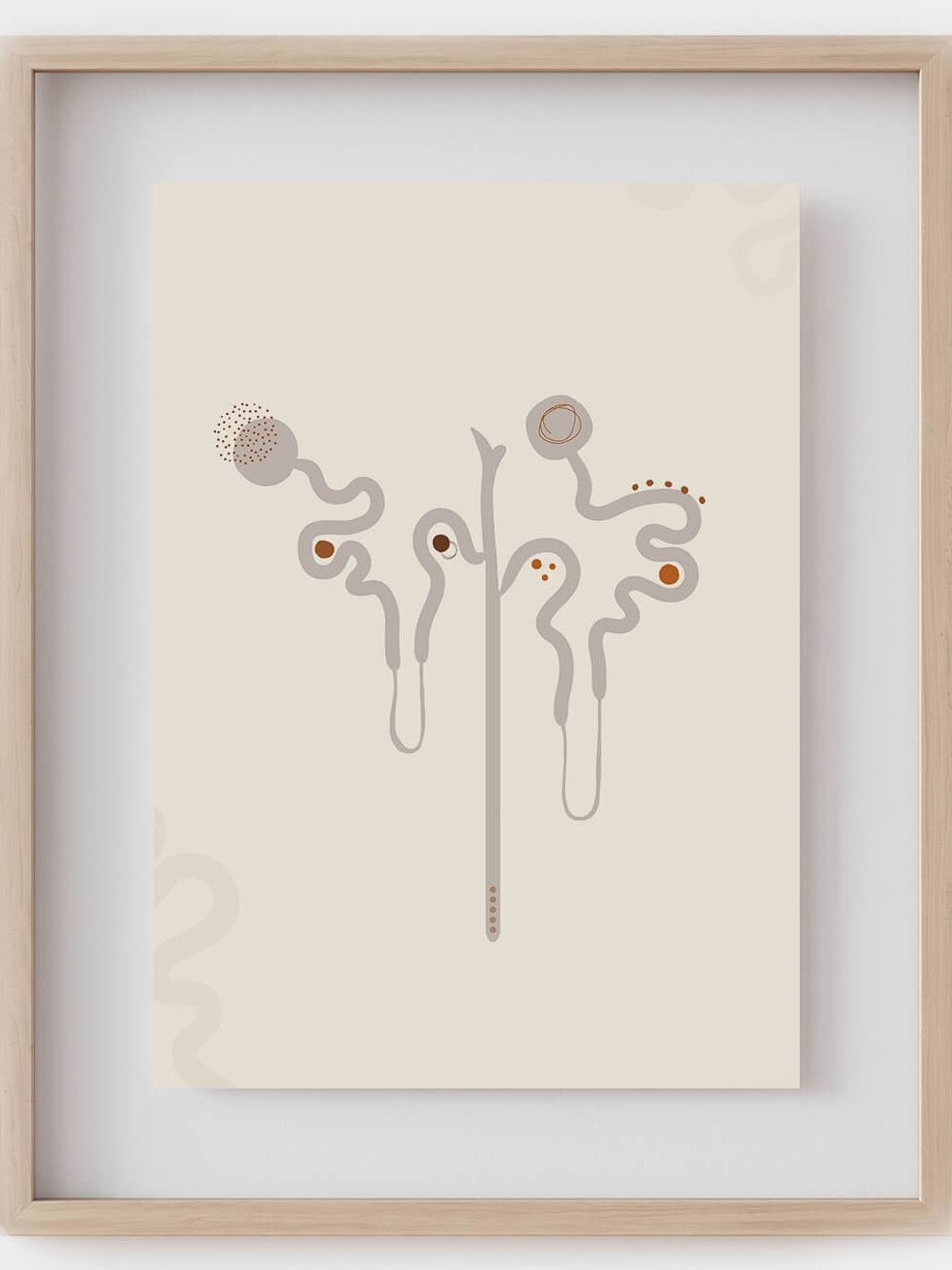The artwork, meticulously framed within clear glass bordered by light wood, is presented on a pristine sheet of white paper. At the heart of the composition lies a prominent gray line running vertically. From near the top of this central line, delicate squiggly lines extend outward symmetrically, each gracefully arching downward before rising up again. Topping off these lines are round gray circles. 

On the left side, maroon dots are meticulously clustered above the gray circle, with additional dots nestled in the bends of the squiggly lines. The circle on this side is uniquely marked by a smaller maroon circle within it. Further maroon dots are thoughtfully scattered along the squiggly lines, as well as adorning the lower portion of the central stem line.

Adding to the complexity, the lower left and the upper right corners feature lighter gray squiggly lines, lending a balanced and harmonious feel to the entire composition.